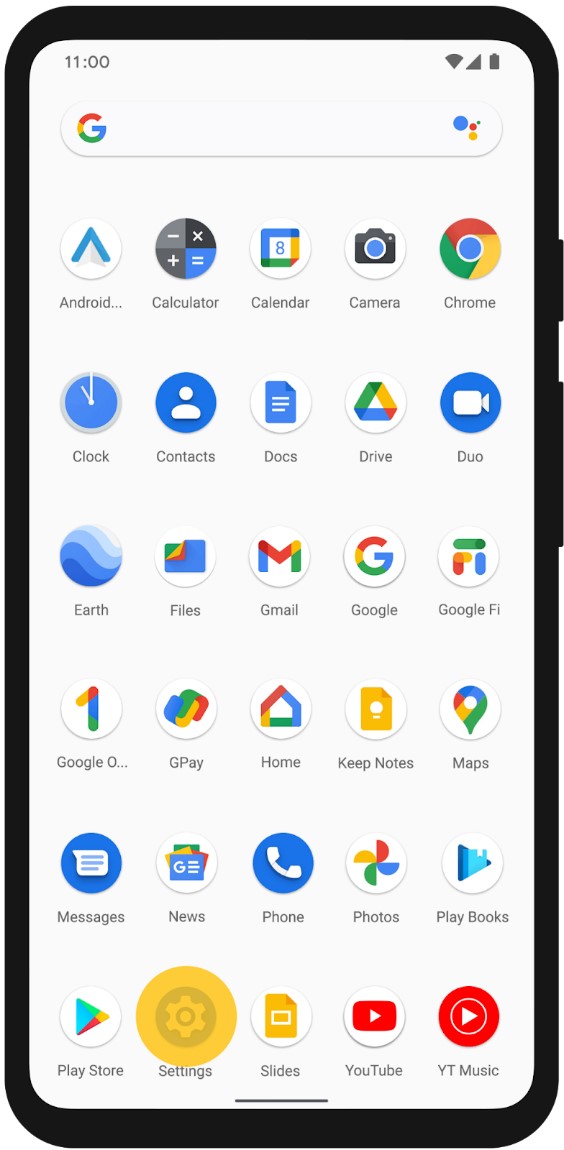The image depicts a mobile device with a sleek black frame. On the upper right side of the device, a black power button is visible, with volume up and down buttons located just below it. The screen, set to a white background, displays the app section featuring several rows of installed apps. At the top of the screen, there is a Google search bar. 

In the first row of apps, we can see icons for Google, Calculator, Calendar, Camera, and Chrome. The second row features Clock, Contacts, Docs, Drive, and Duo. Moving to the third row, the icons displayed are for Earth, Files, Gmail, Google, and Google Fi. The fourth row shows apps like Google One, GPay, Home, Keep Notes, and Maps. 

In the fifth row, the icons include Messages, News, Phone, Photos, and Play Books. Finally, the sixth row consists of the Play Store, Settings, Slides, YouTube, and YouTube Music icons. Each app icon is neatly arranged, showcasing the organizational layout of the device's home screen.